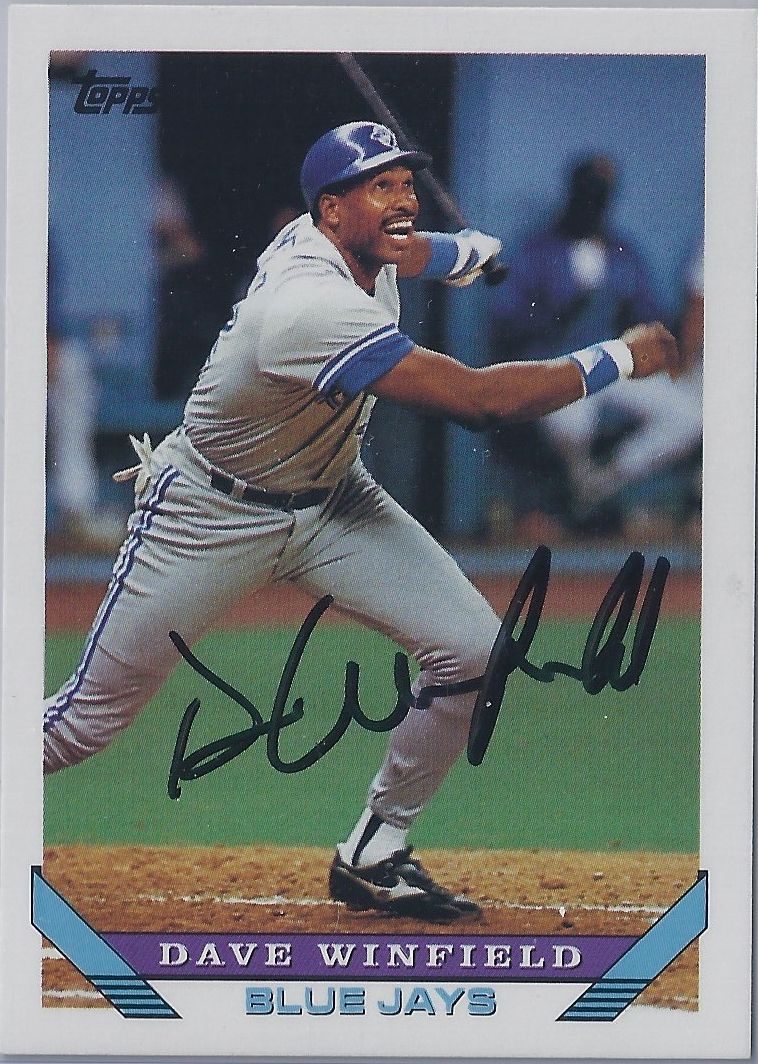This is an image of a rectangular baseball card by Topps with "Topps" written in the upper left corner. The card features a gray border, and in its center, there is a dynamic picture of a Black baseball player standing in the batter’s box. The player, Dave Winfield, is shown right after taking a swing, with his black bat extended in his left hand behind him. He is wearing a mostly gray uniform with white and blue stripes down the legs, a blue t-shirt under his jersey, blue and white wristbands, and a dark blue batting helmet adorned with the Toronto Blue Jays logo. His face is turned upward in a smile, revealing his teeth. Behind him, the background is blurred but includes indistinct images of people and the infield. At the bottom of the card, it reads "Dave Winfield" in white text and "Blue Jays" in blue text, with Winfield's autograph across the lower part.